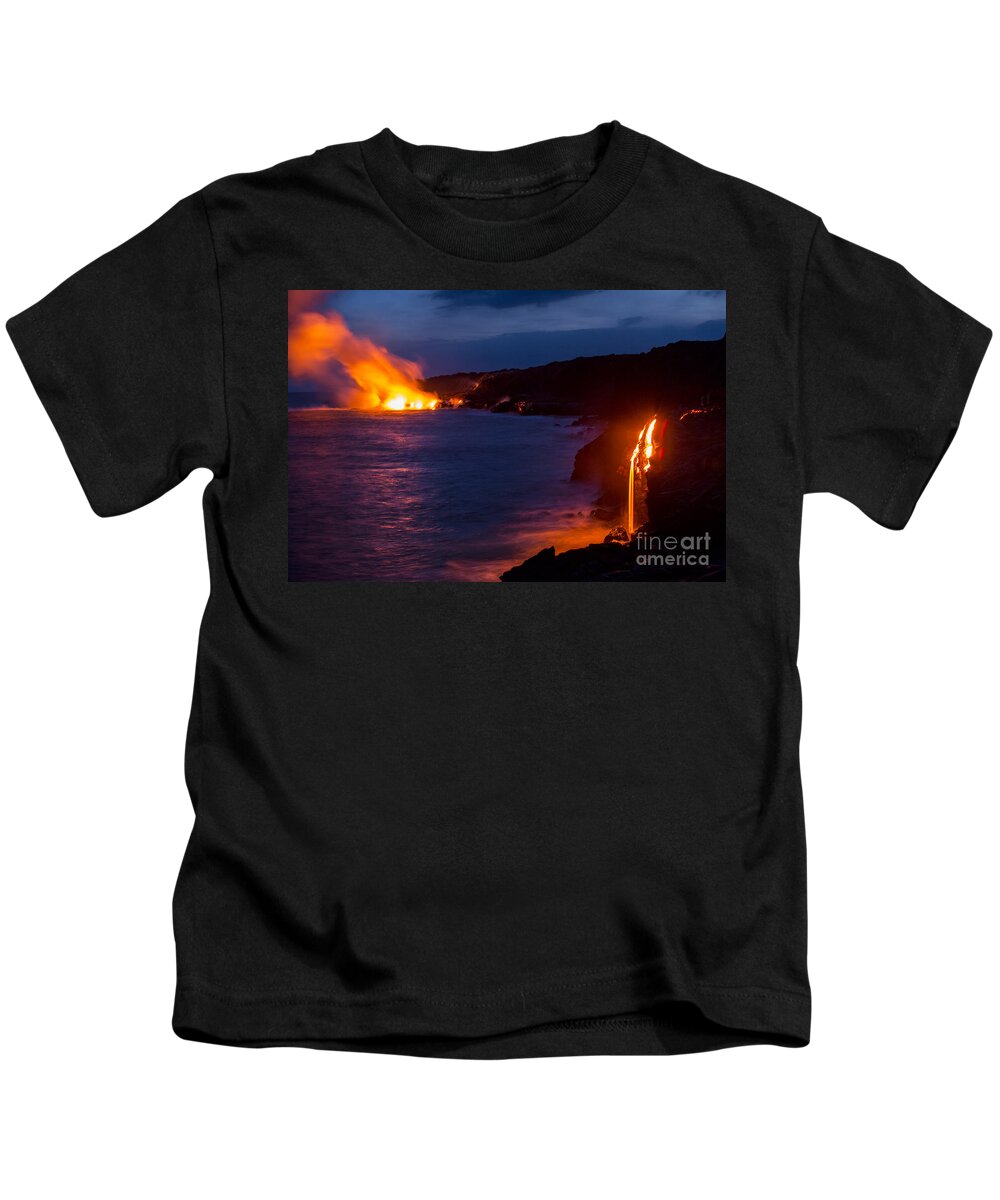The image features a black, unbranded, short-sleeved T-shirt set against a stark white background. Prominently displayed across the chest of the T-shirt is a rectangular graphic depicting a dramatic volcanic landscape. The scene captures a hilly landmass with molten lava cascading down into a body of water, creating a striking visual contrast. On the right side of the graphic, lava appears to fall like a waterfall into the water, causing a noticeable reaction as steam and smoke rise into the air. In the background, there are dramatic flares and larger eruptions, with fire visibly burning on top of the landmass and smoke rising above it. The sky above the scene is a dark, almost foreboding blue, interspersed with grayish-white clouds. The bottom right corner of the graphic bears the small gray-white text "Fine Art America."